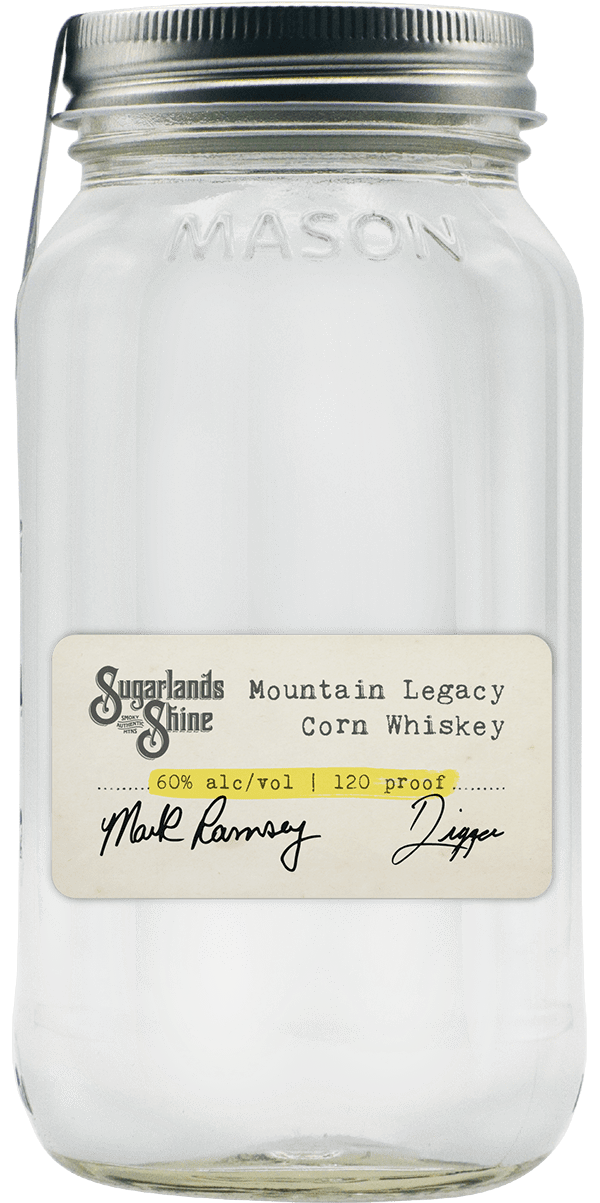The image features a clear glass mason jar with a wide body and a silver aluminum twist cap. The word "mason" is embossed near the top of the jar. The front of the jar has a crisp white rectangular label prominently displayed halfway down. The label bears the text "Sugarlands Shine," which appears as a professional logo. Below this, in a serif font, are the words "Mountain Legacy Corn Whiskey." Highlighted against a subtle yellow background, the label specifies the contents as "60% alcohol volume / 120 proof." There are black cursive signatures underneath, reading "Mark Ramsey" and "Digger." The backdrop of the image is plain white, suggesting it was shot in a professional setting without any additional text or website information present. The overall color scheme includes black, white, clear gray, silver, and yellow.